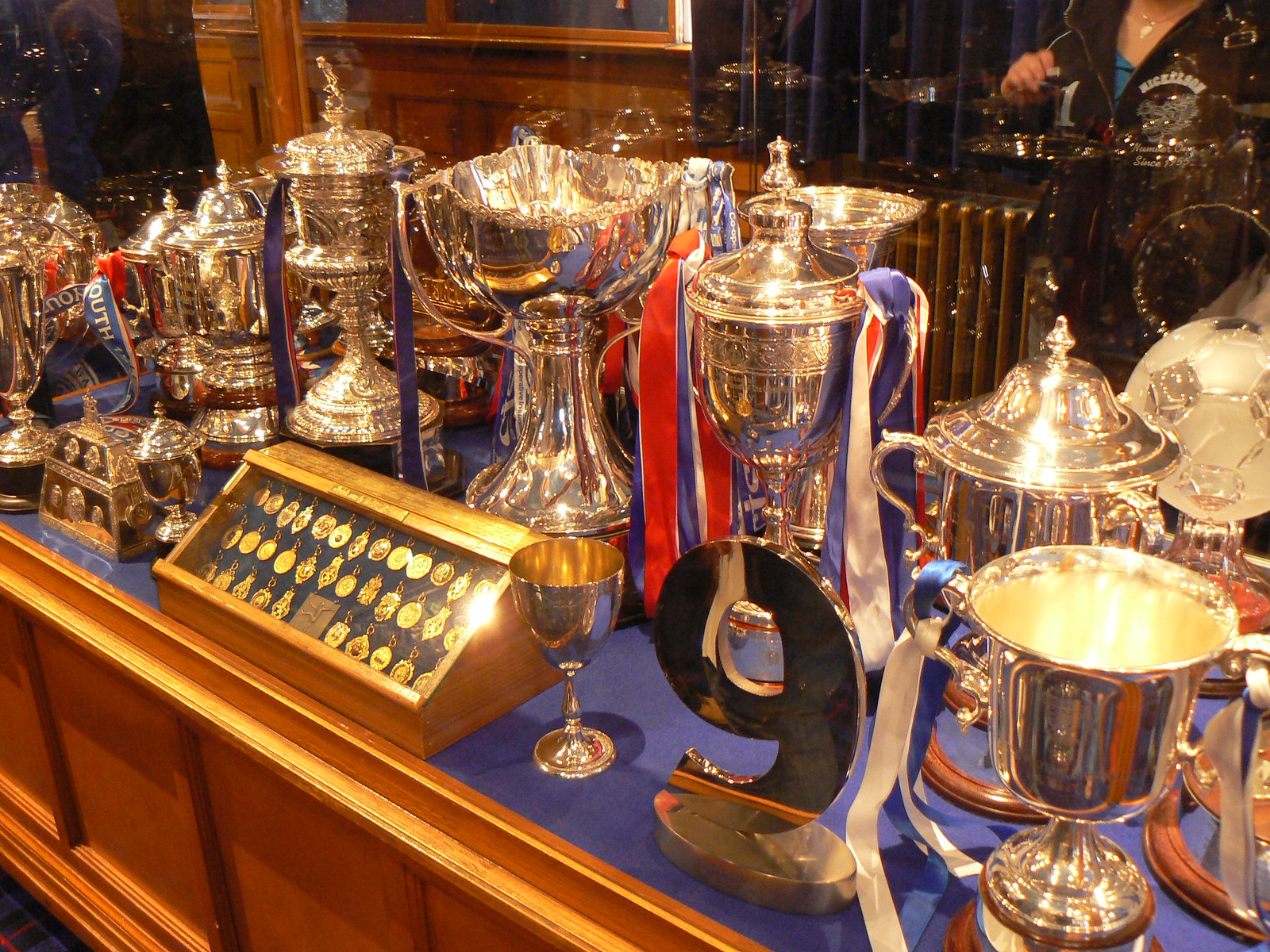This is a high-quality color photograph of a wooden display case featuring a diverse array of trophies and medals. The trophies, predominantly gold and sizable cup trophies similar to those awarded in prestigious tennis tournaments like the French Open, are meticulously arranged inside the case. Some of the prominent trophies have large gold "9" figures and a few have silver variants adorned with hanging ribbons. The display case has a plush, bluish velvet-lined base, and a pristine glass front, which captures the reflection of a woman wearing a black track jacket with writing on it. In the foreground, the light gleams off the gold trophies, enhancing their lustrous appearance. Additionally, smaller gold medals, likely intended to be worn around the neck, are visible, further adding to the impressive collection housed within the elegant wooden and glass cabinet.